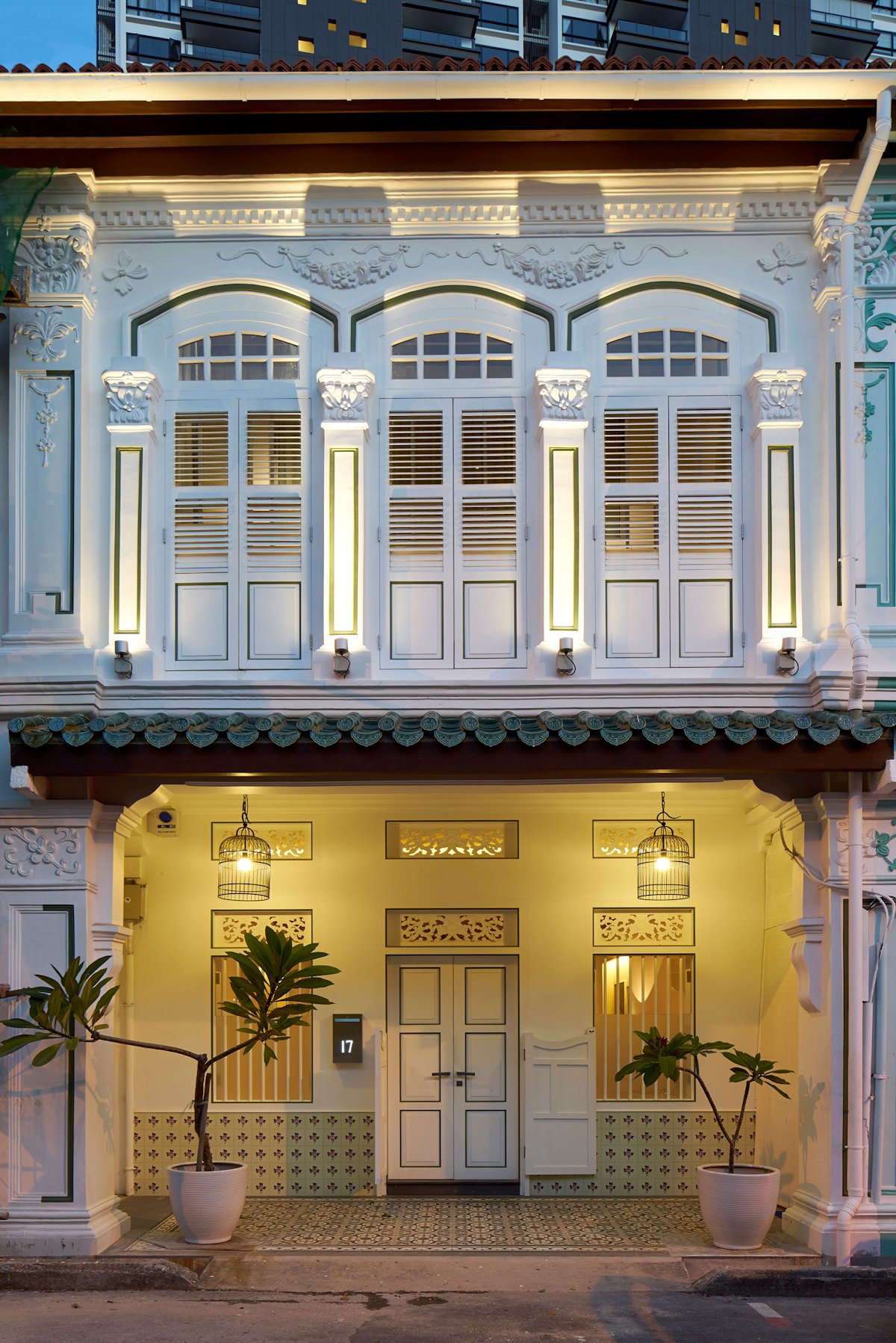This image showcases the front facade of an elegant, two-story building, possibly an apartment or small hotel, captured from a street-level view. The structure is predominantly white, adorned with intricate, French-inspired details. The lower level features a double-entry door flanked by two potted plants, one on each side, set in large, white planters. Above the door, there is a prominent number "17" displayed on a mailbox. 

Twin lamps hang from the ceiling, casting a warm, yellow light that suggests the photo was taken in the evening. The ground level also includes two windows with patterned designs beneath them. Moving up to the second floor, three additional windows are visible, separated by four ornate white pillars, highlighted by spotlights that cast dramatic shadows. The roof is tiled and green, with further intricate white detailing lining the top.

Additionally, a larger building with several windows and balconies peeks out from behind the structure, signifying the presence of a busier, more urban environment. A gutter downspout is visible on the right side of the building, and the surrounding street is gray, completing this picturesque scene reminiscent of a charming coastal town.